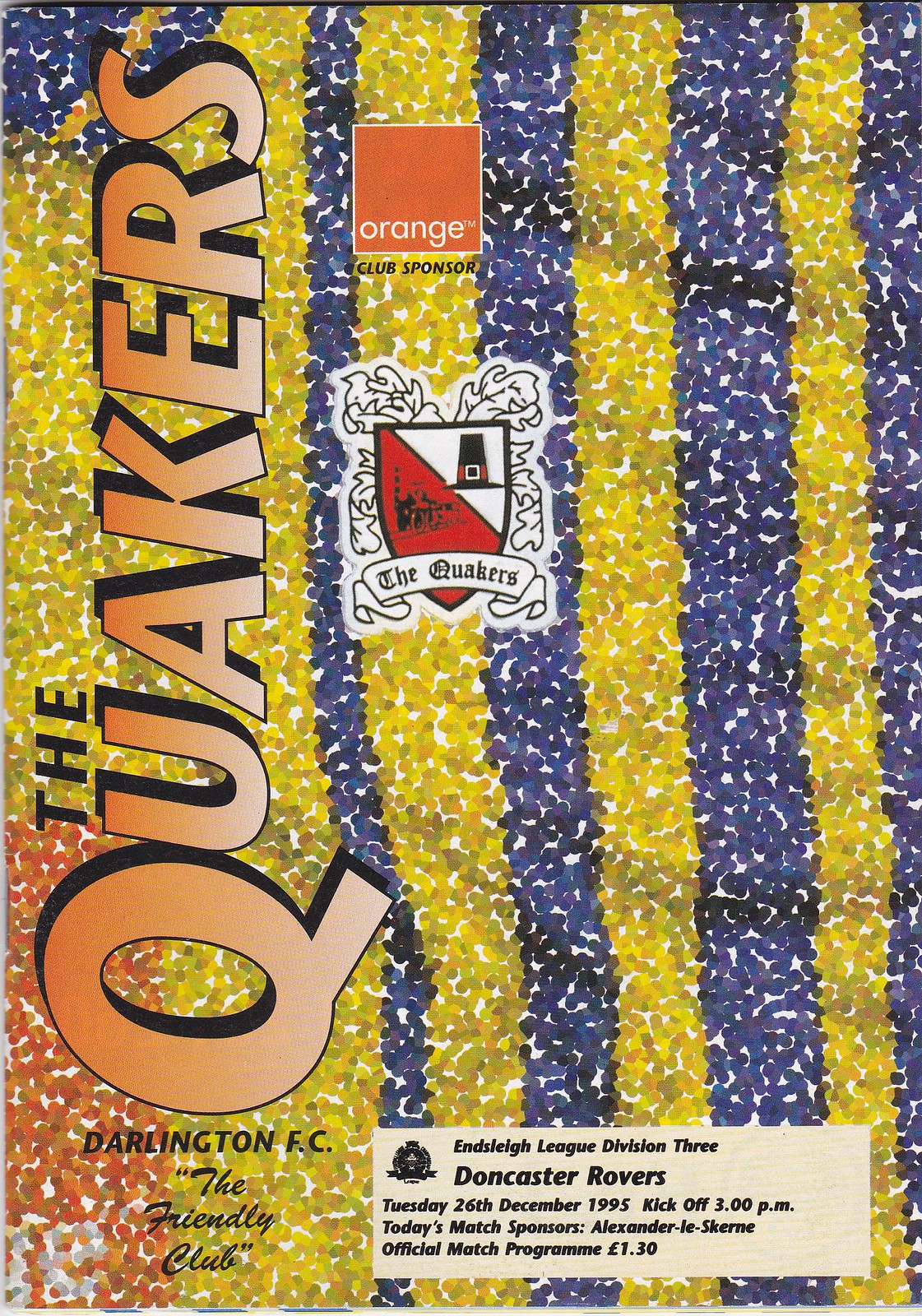The image features the cover of a magazine with a distinctive background consisting of alternating vertical stripes in blue and yellow, created with closely spaced dots that produce an eye-catching pattern. On the left side of the cover, the text "The Quakers" is oriented vertically and rendered with an orange-to-white gradient, outlined in black, requiring a head tilt to read comfortably. To the right of this, set within an orange box, is the phrase "Orange Club Sponsor," displayed in white letters. Below lies a emblematic crest showcasing a shield divided vertically into red and white sections, adorned with a Quaker hat and leaves behind it. Central to the image, the logo prominently features the text "The Quakers." At the bottom, the details of a sporting event are meticulously noted: "Darlington FC, The Friendly Club, Slay League Division 3, Doncaster Rovers, Tuesday 26th December 1995, kickoff 3 p.m.," alongside "Today's match sponsors: Alexander Lasker" and "Official match program: €1.30."